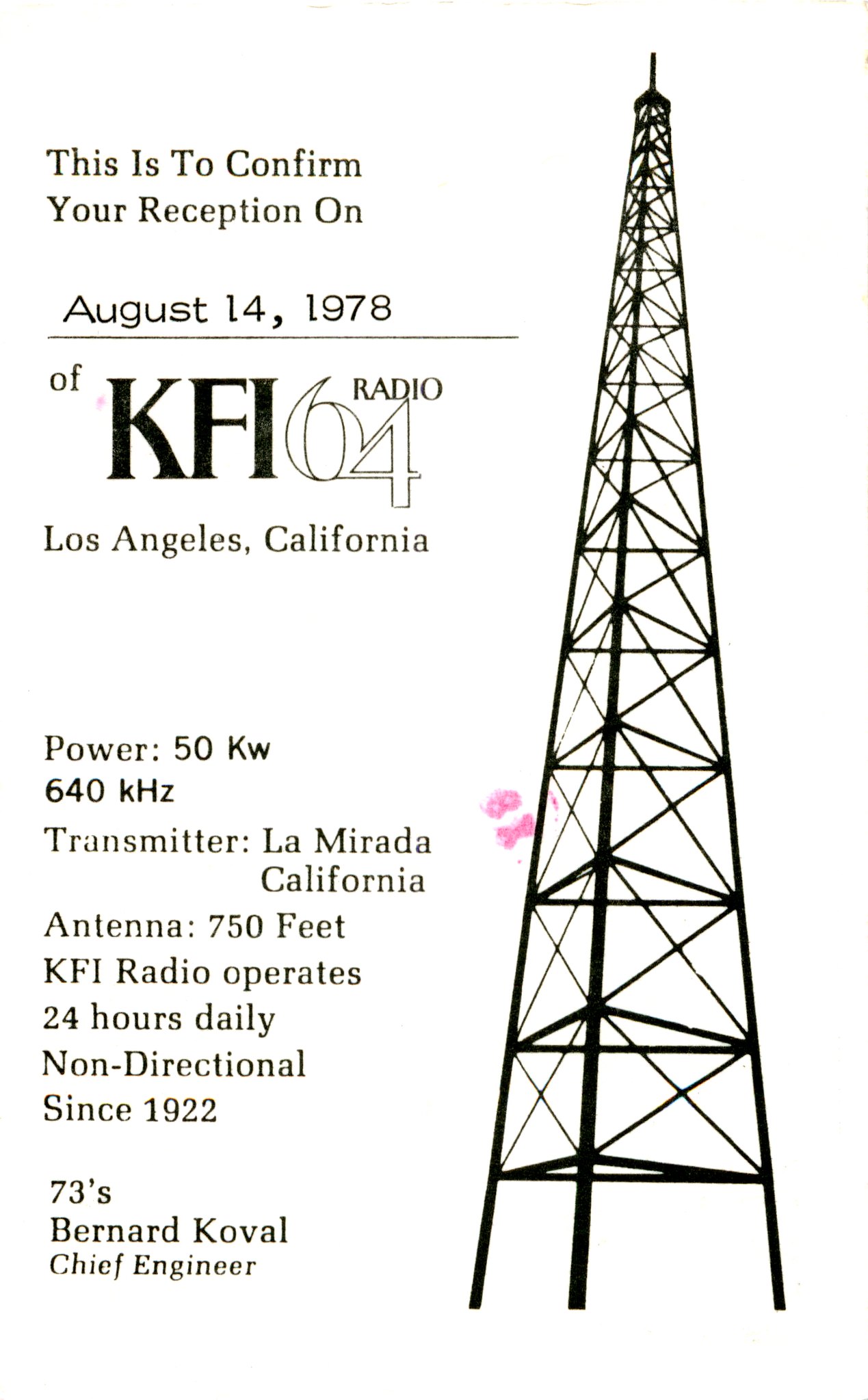This black and white image is a confirmation notice for the reception of KFI-64 radio in Los Angeles, California, dated August 14, 1978. The right-hand side of the image features a detailed illustration of a radio tower. The left-hand side is filled with descriptive lettering. Notably, just beneath the "LA" section, the power specifications are listed, including the kilowatts and kilohertz of the transmitter located in La Mirada, California. The notice also states that the antenna is 750 feet tall, and that the radio station has been operating 24 hours a day, non-directional, since 1922. Beneath this detailed information, the image is signed off with "73's Bernard Covel, Chief Engineer."